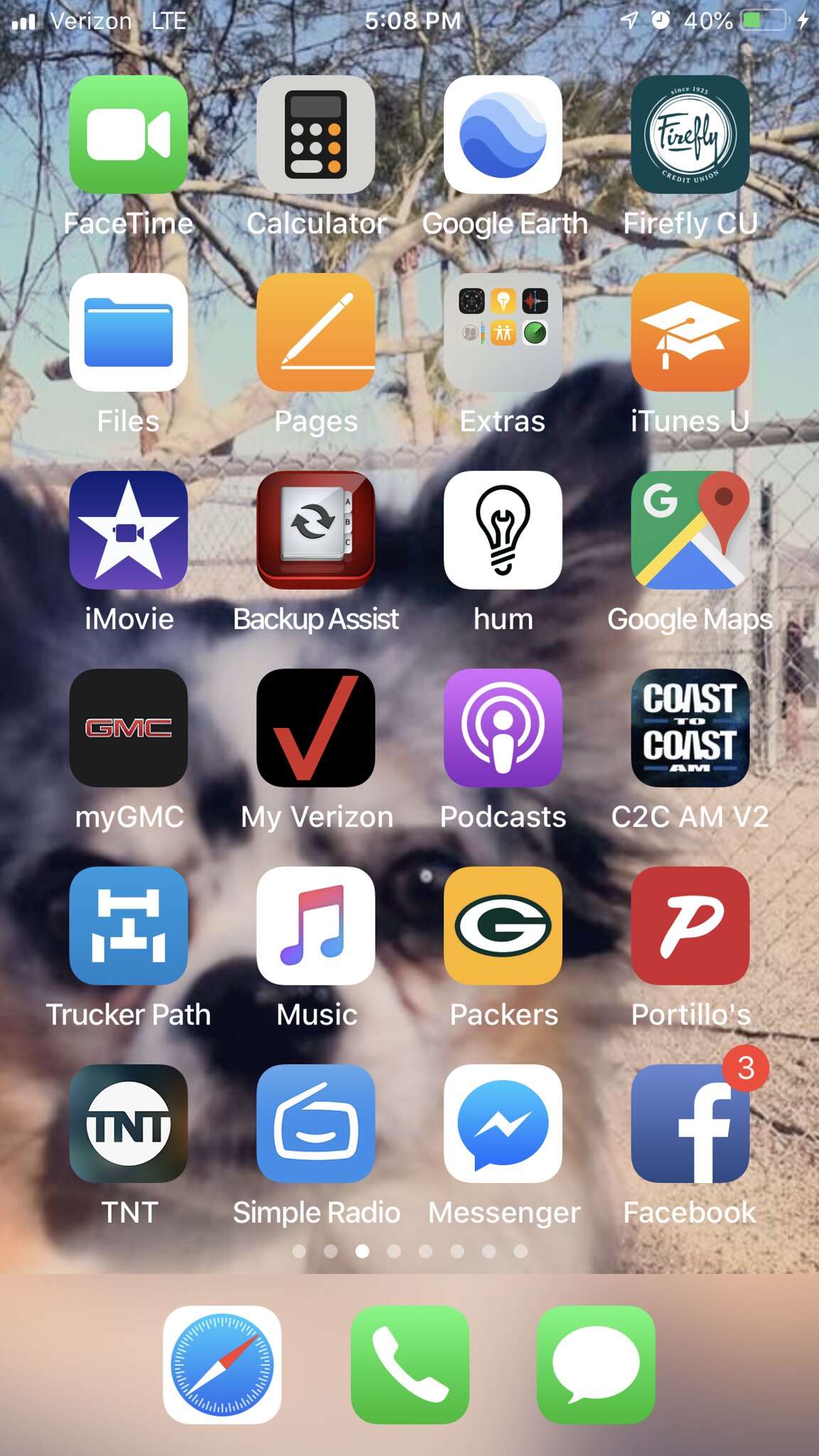This detailed screenshot showcases a smartphone's home screen with various app icons organized across seven rows of four apps each, except for the last row which contains three apps. Here's a comprehensive breakdown of the home screen elements:

- **Status Bar:**
  - Top left: Three internet bars indicating connection strength.
  - Going right: "Verizon LTE" indicating the carrier and network type.
  - Center: Current time displayed as 5:08 p.m.
  - Right side: An alarm clock icon signaling a set alarm, and a battery icon showing 40% charge remaining.

- **App Layout:**
  - **First Row (Left to Right):**
    - FaceTime
    - Calculator
    - Google Earth
    - Firefly CU

  - **Second Row (Left to Right):**
    - Files
    - Pages
    - Extras
    - iTunes

  - **Third Row (Left to Right):**
    - iMovie
    - Backup Assist
    - Home
    - Google Maps

  - **Fourth Row (Left to Right):**
    - MyGMC
    - MyVerizon
    - MyPodcast
    - C2CAMV2

  - **Fifth Row (Left to Right):**
    - TruckerPath
    - Music
    - Packers
    - Portfolios

  - **Sixth Row (Left to Right):**
    - TNT
    - Simple Radio
    - Messenger
    - Facebook (notable red notification badge with white number "3")

  - **Seventh Row (Left to Right):**
    - A compass icon with a blue background, red arrow pointing up right, and white arrow pointing down left
    - A green square bearing a phone icon diagonally positioned from the top left to bottom right
    - Another green square with a speech bubble icon indicative of messaging

- **Background:**
  - A charming puppy dog looks directly at the camera, framed against a backdrop of blue sky and a tree.

This thoroughly detailed description encapsulates all the elements, providing a clear picture of the smartphone's home screen, its layout, and content.